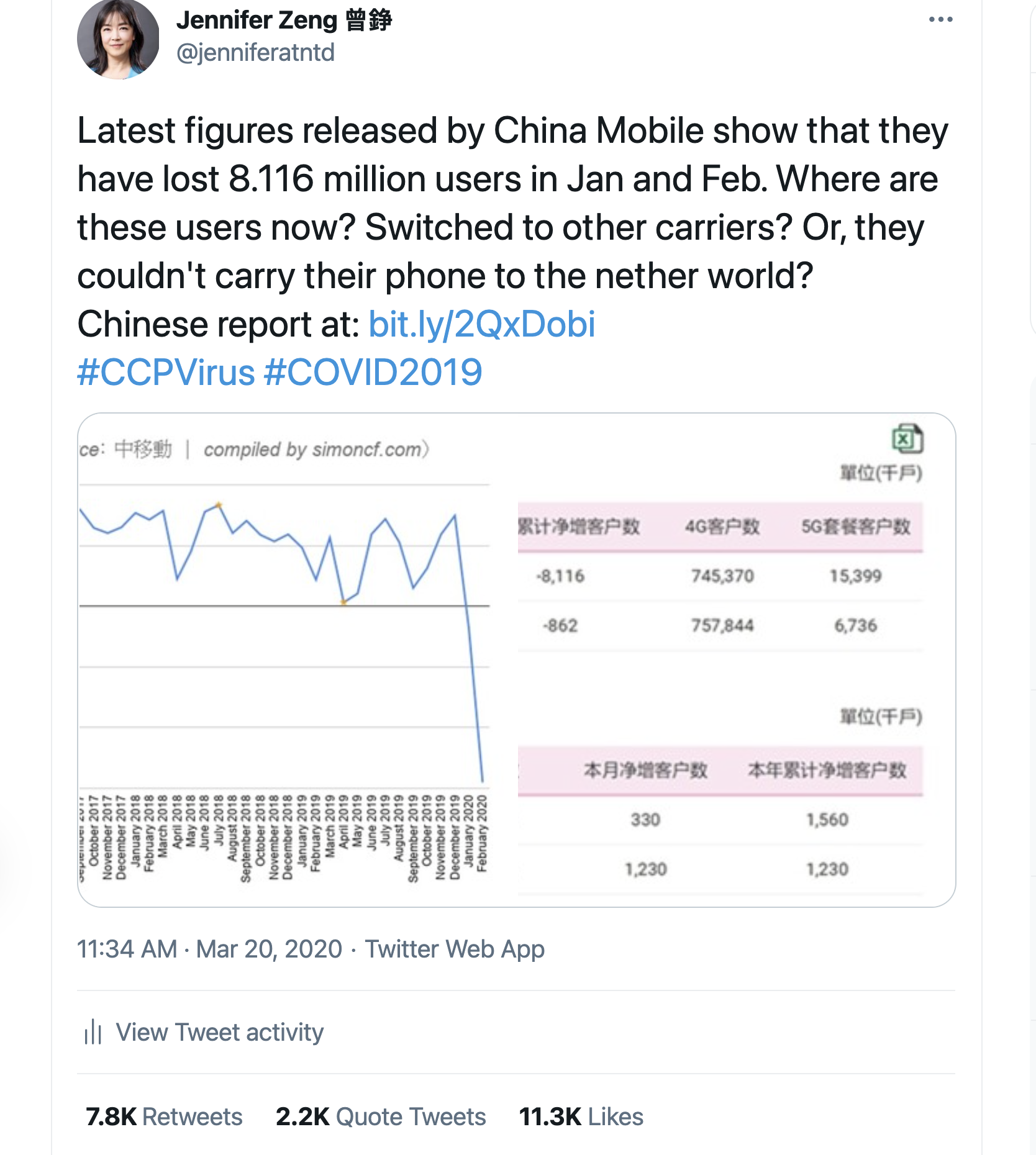**Caption for Social Media Image Description:**

The social media post features primarily black text set against a white background. In the top-left corner, there is a circular profile image of a woman, identified as Jennifer Zeng. She appears to have dark hair and light skin, wearing what seems to be a black jacket or perhaps a blue top. Beside her name are two Chinese characters. In the top-right corner, three dots are visible.

Below the profile image, black text provides an update on recent statistics, mentioning that China Mobile lost 8.116 million users in January and February. The text questions whether these users switched to other carriers or if their inactivity could be attributed to more dire circumstances, implied by the phrase "couldn't carry their phone to another world." 

There is a link to a Chinese report (bit.ly/2qxdobi/ccpvirus) followed by hashtags: #ccpvirus and #COVID-19, hinting that the post is related to the COVID-19 pandemic.

A blue-line graph is situated below this text, accompanied by smaller, nearly unreadable text. To the right of the main graph, two more graphs with Chinese numerals and pink-highlighted rows depict supplementary data. 

At the bottom of the post, the timestamp "11:34 AM March 20, 2020" is visible, along with Twitter-related metrics including "Twitter Web App," "YouTweet activity," "7.8k retweets," "2.2k quote tweets," and "11.3k likes." This data suggests significant engagement, reinforcing the post's importance and relevance.

The commentary centers on the COVID-19 pandemic, questioning the disappearance of millions of users from China Mobile's network during the early months of 2020.